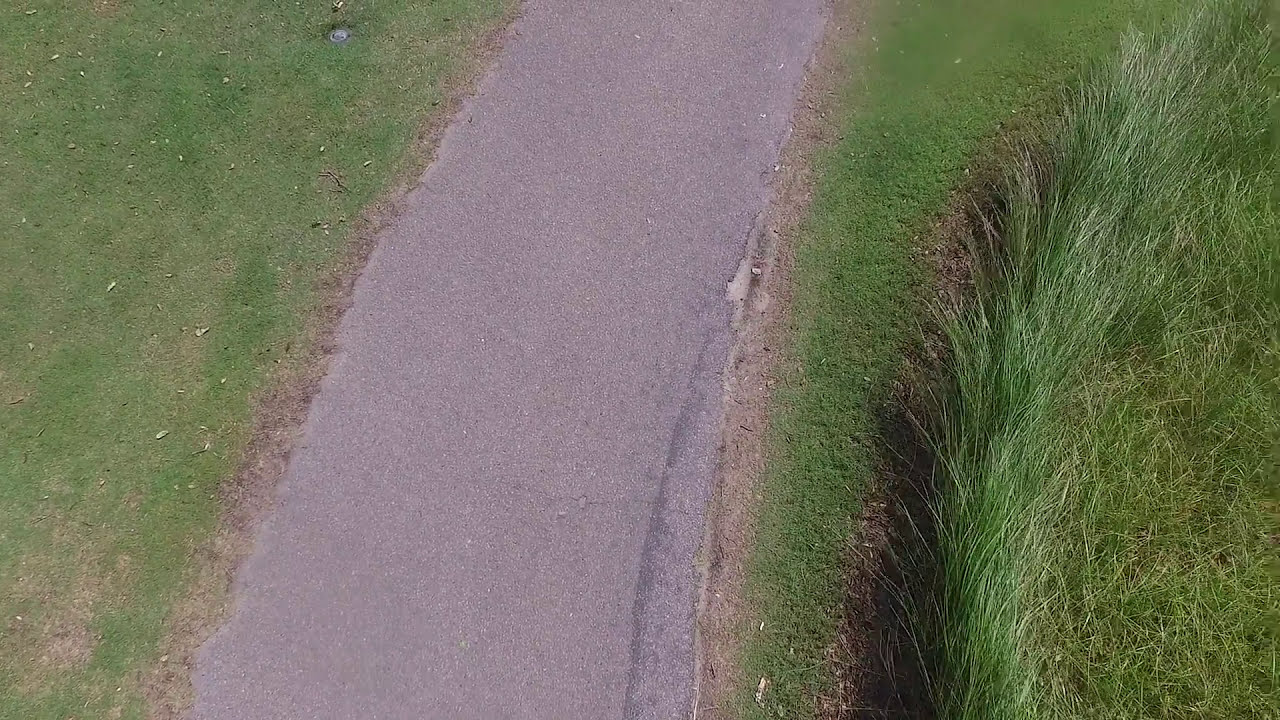This aerial photograph, likely taken from a low-altitude drone, showcases a gently curving, light gray path or walkway that extends from the bottom left to the middle top of the image. The path has no shoulder or lines, emphasizing its natural integration with the surrounding environment. On both sides of the path, there is short green grass, which transitions into taller, flowy grass as you move rightward across the image. Shadows cast by this tall green grass create striking contrasts on the ground, indicating a sunny day. On the far right side of the photograph, the tall grass suggests proximity to water. Additionally, the top left of the image features a small, rounded gray object nestled in the grass, distinct from the surrounding foliage but too small to be easily identified. The scene is devoid of any human or animal presence, enhancing the serene and undisturbed quality of this park area.